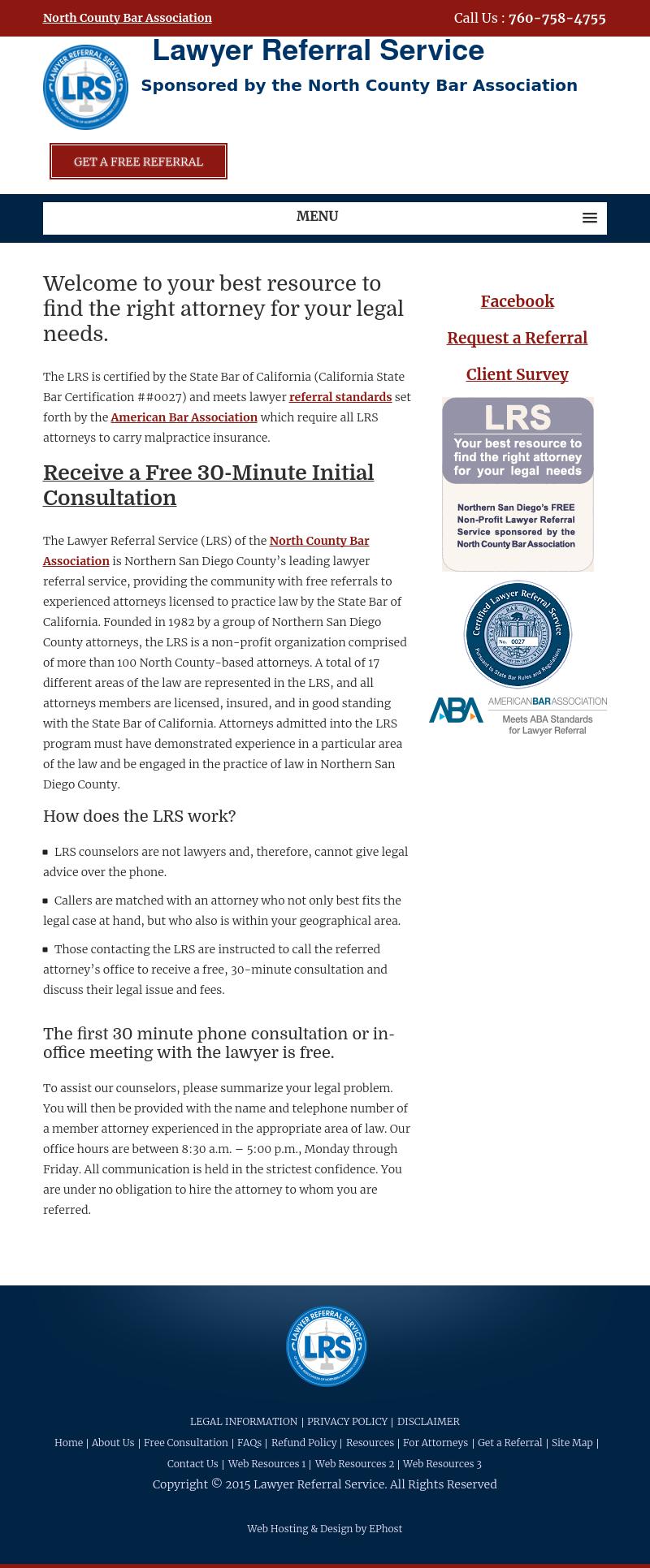In this screenshot of a website, a prominent red header at the top displays "North County Bar Association." On the upper right corner, the text "Call us: 760-758-4755" is visible. Below the header, in blue text, it reads "Lawyer Referral Service, sponsored by the North County Bar Association," with a blue circle showcasing the initials "LRS." Beneath this, a red action button labeled "Get a Free Referral" stands out. Underneath the button, a white bar with the word "Menu" is present. The main section of the webpage features a welcoming message: "Welcome to your best resource to find the right attorney for your legal needs." It also states, "Receive a free 30-minute initial consultation." 

An explanatory section follows with the heading "How does the LRS work?" It clarifies that "LRS counselors are not lawyers and therefore cannot give legal advice over the phone." The text explains that "Callers are matched with an attorney who not only fits the legal case at hand, but who also is within your geographical area." Additionally, "The first 30-minute phone consultation or in-office meeting with the lawyer is free."

At the bottom of the screenshot, it is noted that the web hosting and design are provided by EP Host.